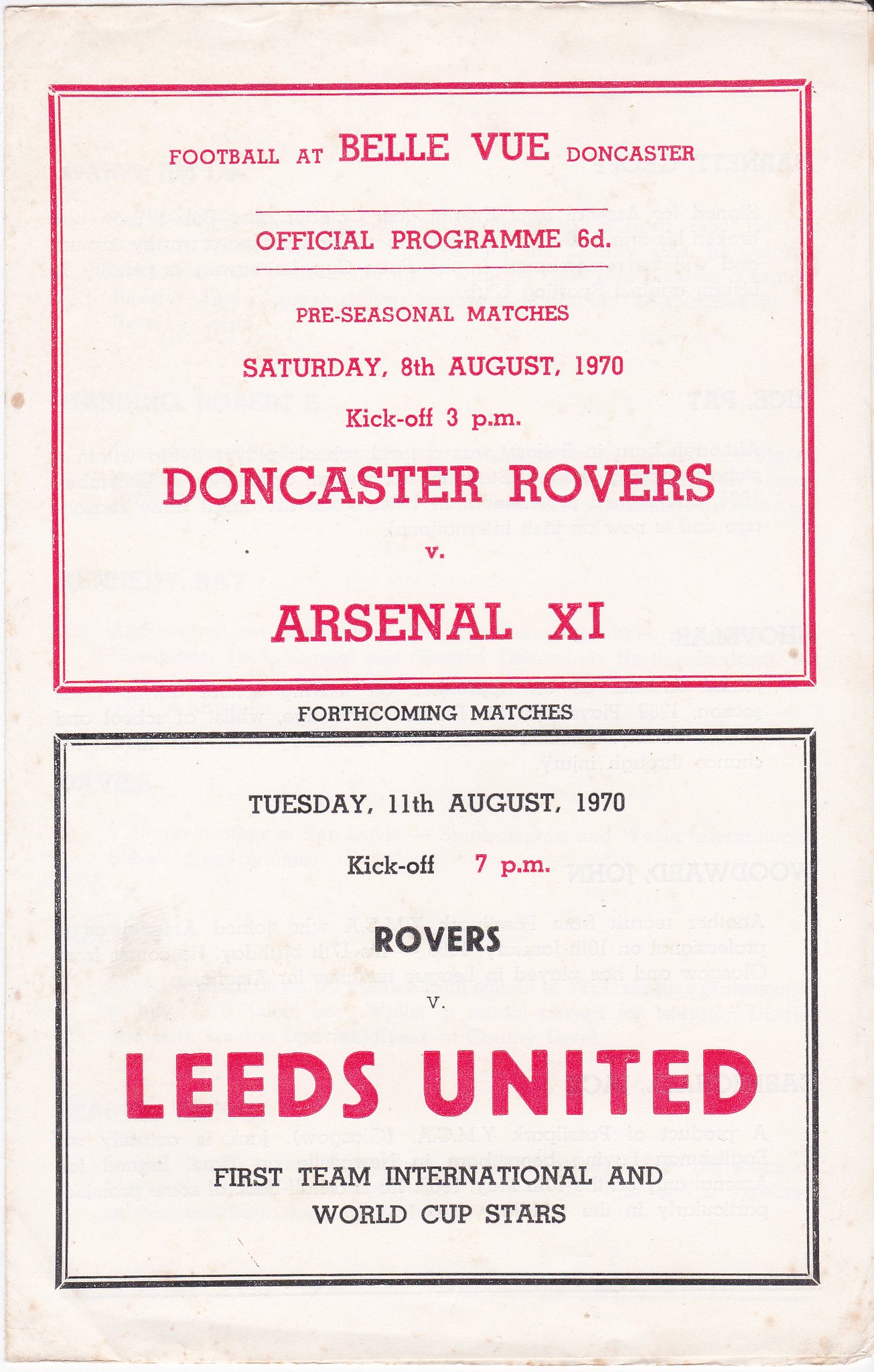The image is a scan of a classic official football program from Bellevue, Doncaster, for pre-season matches dated 1970. The white page, aged and featuring black and red print, displays two main sections. The upper section has a red box with the heading "Football at Bellevue, Doncaster" in red letters. Below that, in smaller black letters, it says "Official Programme" with the British spelling "P-R-O-G-R-A-M-M-E" and a price of "6d" (six pence). The details of the first match are listed: "Pre-seasonal matches, Saturday, 8th August, 1970, kickoff 3 p.m., Doncaster Rovers versus Arsenal XI" in bold red block letters.

The section below this red box, within a black outlined box, is headed by "Forthcoming Matches." It lists the next match scheduled for "Tuesday, 11th August, 1970, kickoff 7 p.m." The text mentions "Rovers V" in small black letters followed by "Leeds United" in bold red letters. Beneath this, it states "first team international and World Cup stars," indicating the prominence of Leeds United during that era. The reverse side of the scanned page shows some text bleeding through, adding to the vintage look of the document.